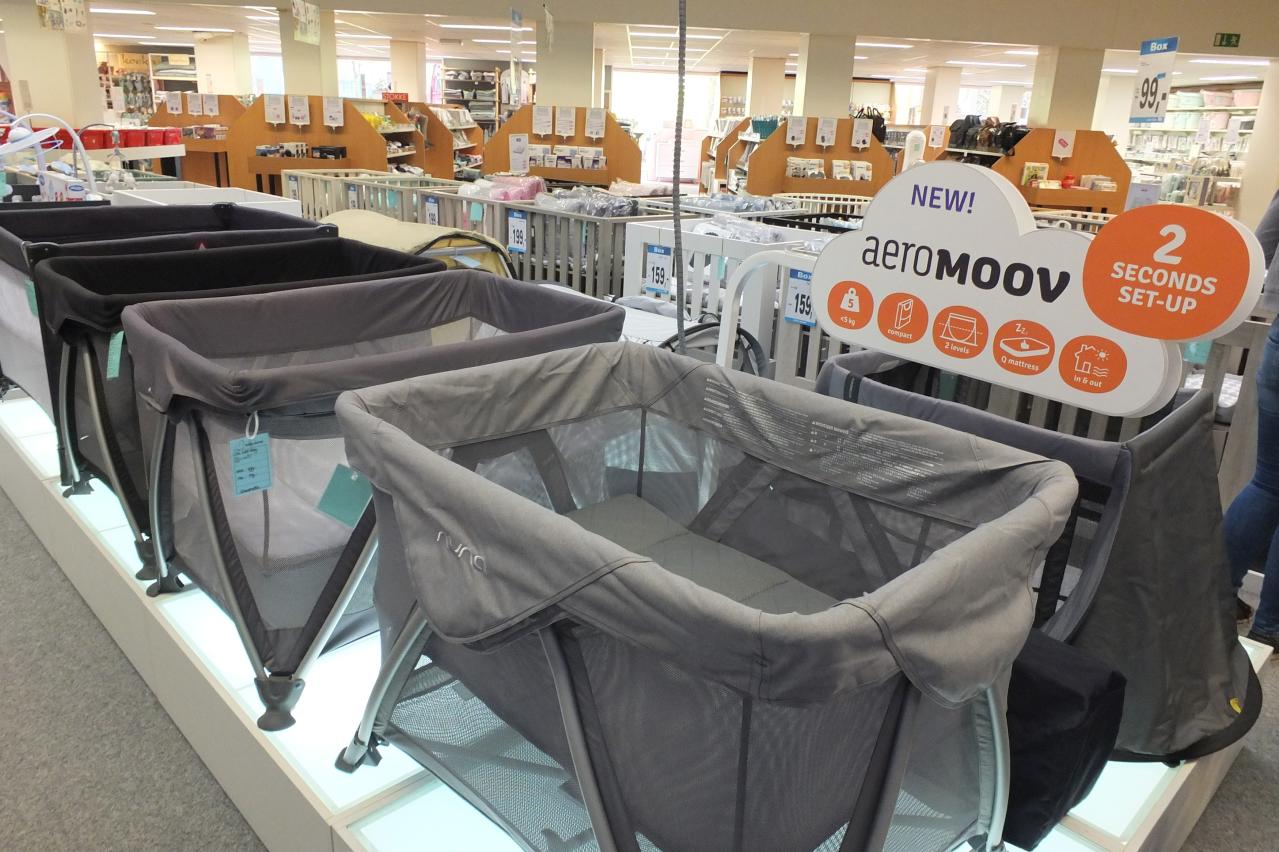The image captures an indoor daytime scene inside what appears to be a department store or a specialized crib store. The focal point is a display of fully assembled baby cribs positioned prominently in the center of the image. These cribs are showcased on a small platform that is illuminated from underneath, adding a distinct glow to the setup. A notable feature is a white cloud-shaped sign on the far right of the display that reads "New AeroMoov" in large letters. The sign also has a large orange circle at the top right with the text "Two seconds to set up," and displays various orange bubbles.

Surrounding the central crib display are various shelves, counters, and bins. The bins appear to contain individually wrapped bedding, each tagged with prices. Shelving units filled with different products are visible in the background, further indicating the retail environment. The carpet flooring adds a uniform texture to the ground. Additionally, windows placed along the top of the image allow natural light to enhance the overall brightness of the store interior. The color palette of the image includes gray, white, light blue, green, orange, red, brown, blue, and purple, offering a visually rich scene.